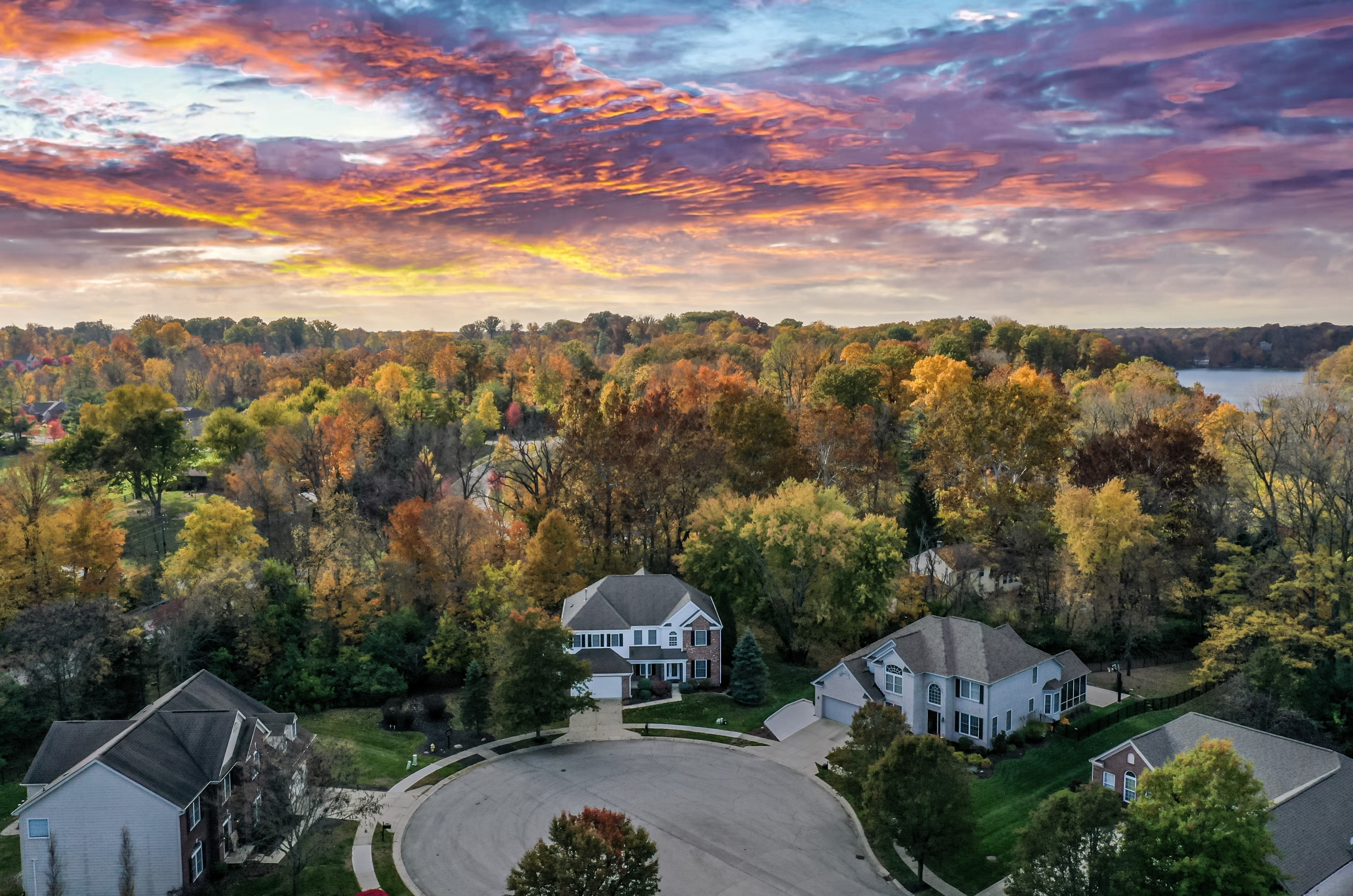This captivating drone shot captures a serene cul-de-sac nestled in a peaceful neighborhood, surrounded by lush greenery and vibrant colors. The composition is thoughtfully structured, with the cul-de-sac and its houses prominently featured in the bottom third of the image. The houses are situated with one directly above the cul-de-sac, two in the top right, and one in the bottom left, each with driveways leading to the gray concrete street.

In the middle third of the image, a dense forest of trees in varying shades of green and yellow dominates the scene, creating a rich, natural backdrop that extends towards the lake located in the top right of this section. The colors of the trees add depth and a touch of autumnal warmth to the landscape.

Above this, the top third of the image features a partly cloudy sky at sunset, painted with a beautiful blend of orange, red, yellow, and purple hues, which reflect off the clouds and contribute to the tranquil atmosphere. This picturesque setting, with its tranquil lake, vibrant flora, and colorful sky, evokes a sense of serenity and peacefulness, making it an ideal place to escape from the hustle and bustle of everyday life.